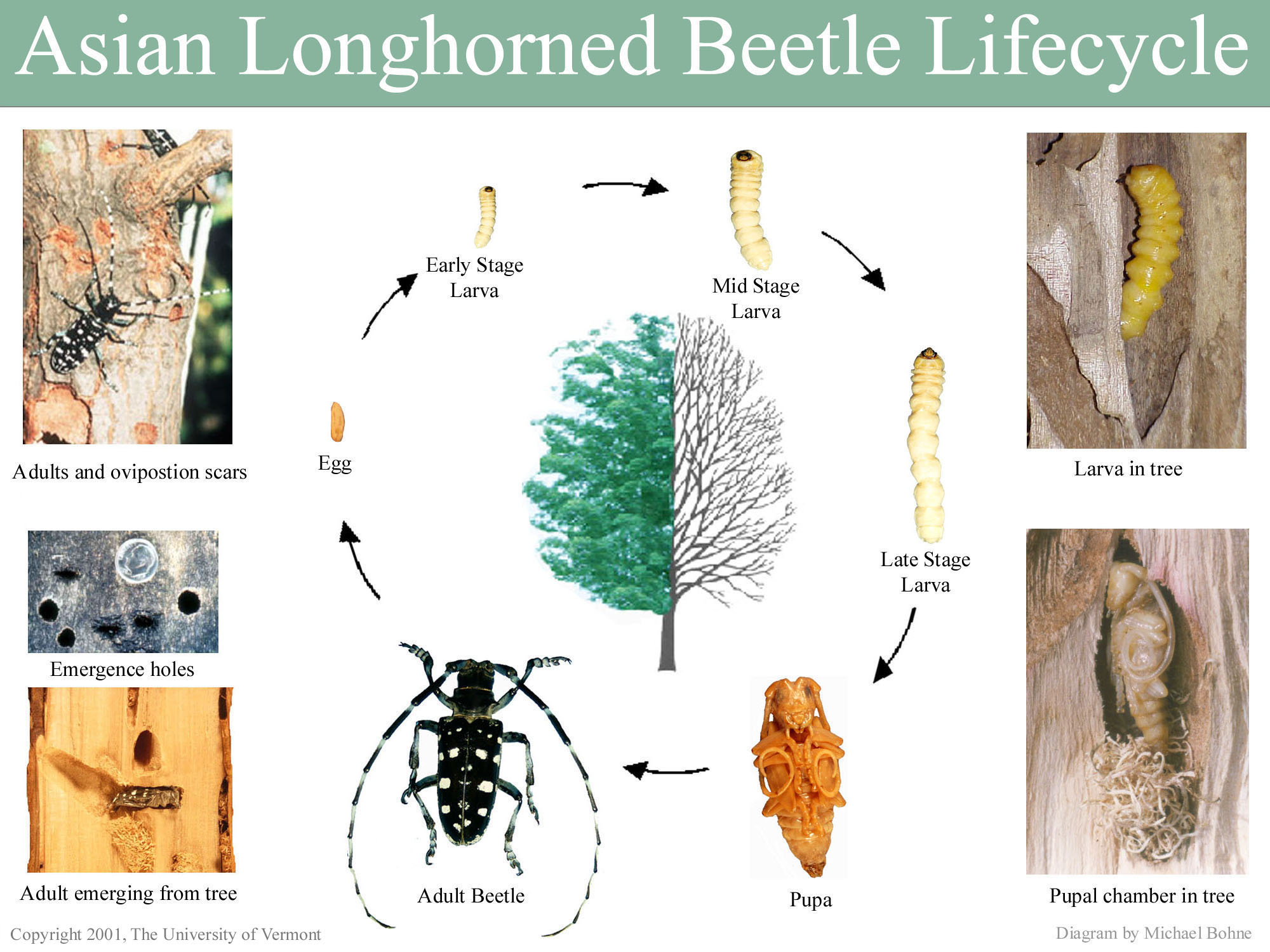This poster, entitled "Asian Long-Horned Beetle Life Cycle," features a sage green banner at the top with white text. Beneath the banner, the poster is divided into three sections showcasing various stages and aspects of the beetle's development. 

On the left side, there are three realistic images: the top image shows a tree with adult beetles and oviposition scars labeled "Adults and Oviposition Scars"; the middle image depicts a tree with emergence holes alongside a dime for size comparison, labeled "Emergence Holes"; and the bottom image shows an adult beetle emerging from a stripped-back piece of wood labeled "Adult Emerging from Tree." 

The central section of the poster features a life cycle diagram with black arrows forming a circular path, illustrating each developmental stage: egg, early-stage larva, mid-stage larva, late-stage larva, pupa, and adult beetle. A visual of a tree accompanies these stages, half with leaves and half barren, representing either the passage of time or the impact on the tree. 

On the right side, two more images are shown: one of the larva inside a tree labeled "Larva in Tree," and another labeled "Pupal Chamber in Tree" detailing the inside of the tree. At the bottom of the poster, it notes "Copyright 2001, University of Vermont," with a diagram credit to Michael Bone.